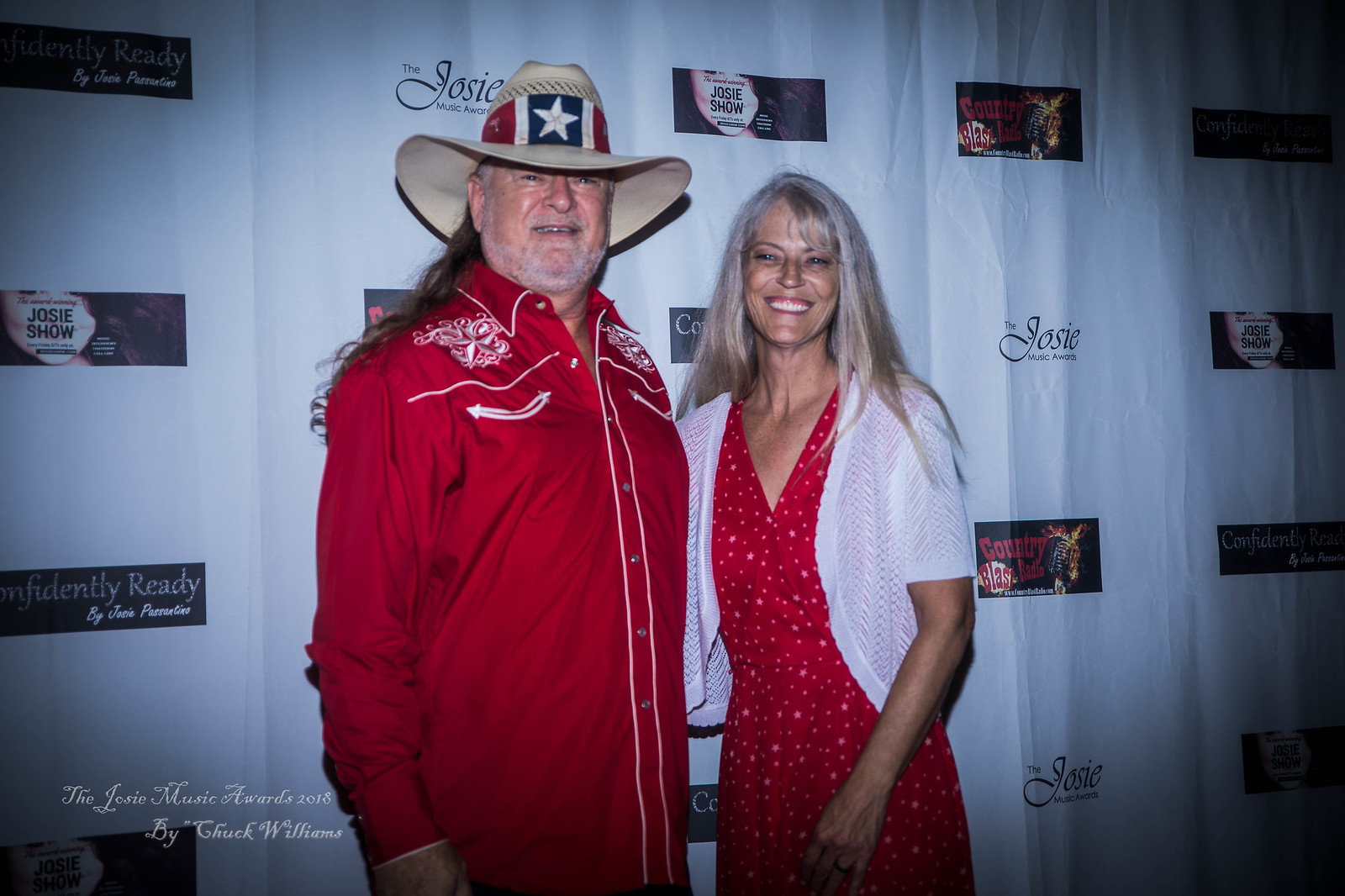The image features a couple, likely nearing retirement age, standing in front of a branded step-and-repeat backdrop adorned with logos for the Josie Music Awards, Country Blast Radio, and Confidently Ready, among others. The gentleman, positioned on the left, is a white male with long curly hair, sporting a cowboy hat embellished with a Texas star and red accents. He has a gray stubble and is dressed in a red button-up long-sleeve shirt, giving off a distinct country western vibe. The lady beside him, positioned on the right, is a slender white female with grey hair. She is wearing a red polka dot dress paired with a white cardigan. Both are smiling warmly at the camera, suggesting they are enjoying their red carpet moment. The backdrop they are standing in front of consists of a white drape featuring various brand logos repeatedly.